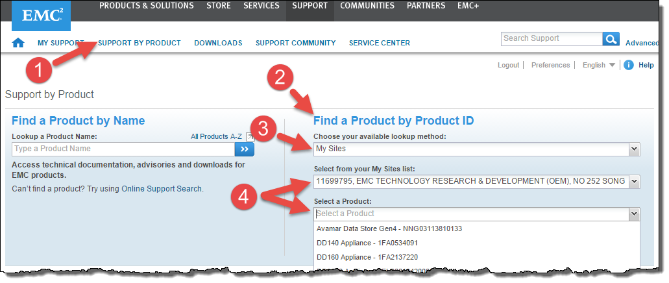The image displays a web page interface from EMC², visually dissected with a torn effect across the middle, which gives the appearance of a ripped page. In the upper left corner, there is a small, bright blue box featuring the EMC logo with "EMC" in white uppercase letters and "squared" in white. A thin black ribbon banner stretches across the top of the page, containing white text with navigational options: "Products and Solutions," "Store," "Services," "Support," "Communities," "Partners," and "EMC Plus."

Below this black banner is a white navigation strip displaying bright blue text. On the far left is a home icon followed by options such as "My Support," "Support by Product," "Downloads," "Support Community," and "Service Center." To the right, there's a short search bar with the placeholder text "Search Support" in gray. Adjacent to the search bar in bright blue text is the word "Advanced."

The primary content area sits on a white background. A filled red circle labeled "1" with white text directs attention to "Support by Product" via a bright red arrow. Further instructions are marked by additional filled red circles: "2" points to "Find a Product by Product ID," "3" indicates "Choose Your Available Lookup Method," and "4" provides dual guidance, pointing to both "Select from Your My Sites List" and "Select a Product," each associated with a dropdown selection. The page clearly illustrates a step-by-step guide on utilizing the support functionalities effectively.